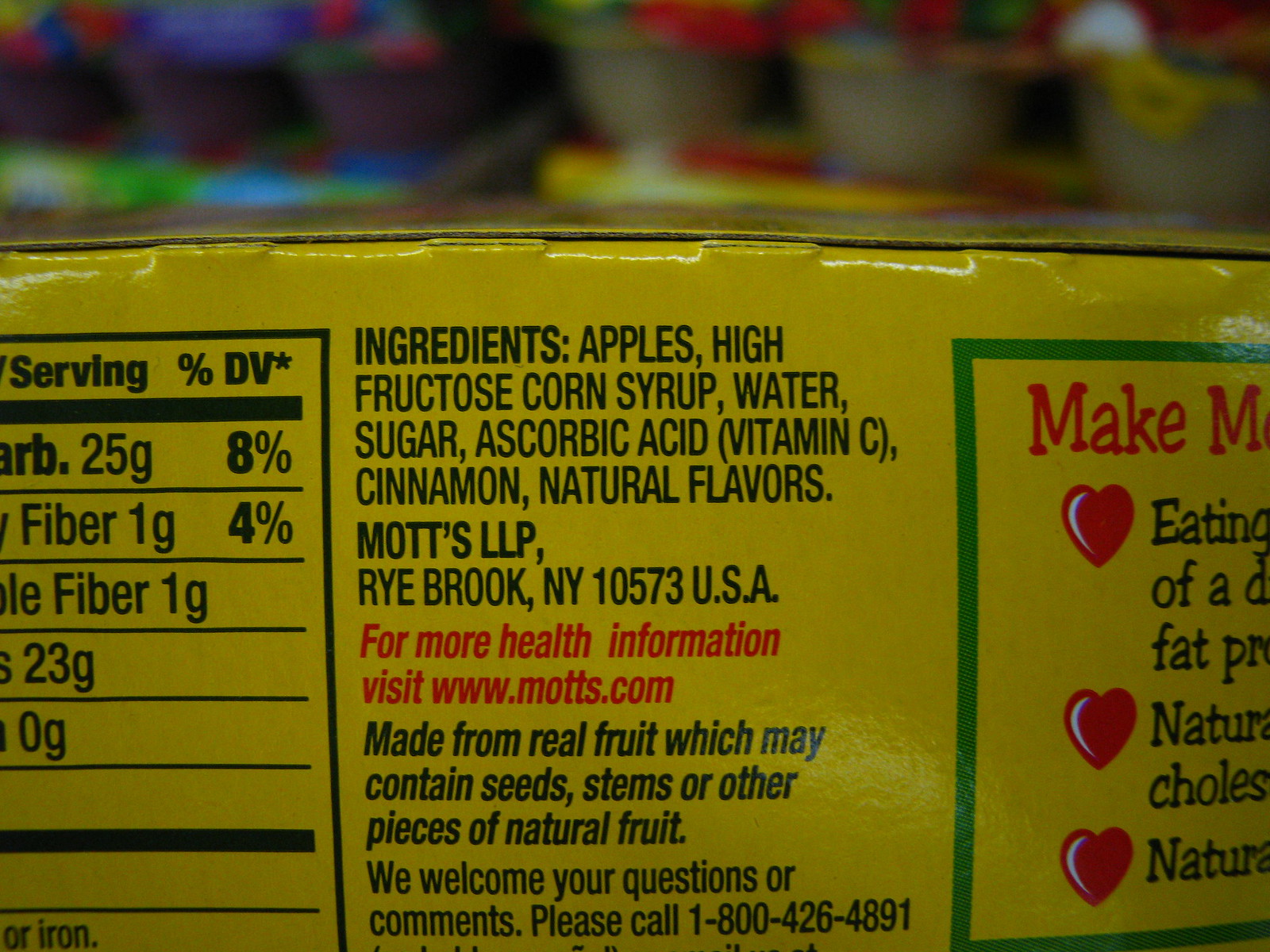A vibrant yellow ingredient label prominently featuring the list of contents: apples, high fructose corn syrup, water, sugar, ascorbic acid (vitamin C), cinnamon, and natural flavors. The central column is dedicated to these ingredients, while the left panel reveals part of the nutritional table. On the right, additional product information, including the manufacturer's details – Mott's LLP, Freiburg, New York, 10573 USA – and a health information website, www.motts.com, are clearly displayed. The label also includes a note that the product is made from real fruit, which may contain seeds, stems, or other natural fruit pieces. Contact information for questions or comments is provided, urging consumers to call 1-800-426-4891. The background is a bright yellow adorned with blurred imagery above, enhancing the visual appeal of the label.